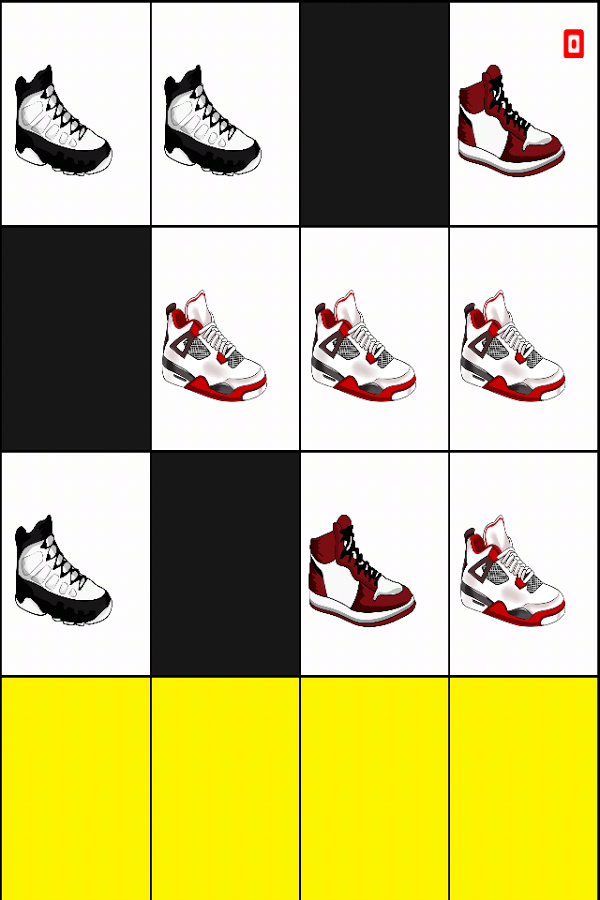The poster is a detailed, grid-layout illustration of various high-top sneakers, arranged in a 4x4 grid for a total of 16 squares. Among these, there are 3 solid black squares and 4 bright yellow squares, all aligned at the bottom row. The remaining squares showcase illustrations of sneakers. The sneakers predominantly come in two color schemes: black and white, and red and white, with a mix of black and white laces. 

1. **Top Row**:
    - The first square features two black and white high-top sneakers with black laces.
    - This is followed by a black square.
    - The third square depicts a white tennis shoe with red and black details and black laces.

2. **Second Row**:
    - The first square presents another black square.
    - The next three squares are identical, displaying white high-top sneakers with red trimming near the toes, red interiors, and white laces.

3. **Third Row**:
    - Starts with a black and white high-top sneaker similar to the ones in the top row, with black laces.
    - Includes another black square.
    - The row ends with two different tennis shoes: one being predominantly white with red and black accents, and the other featuring a mix of red, gray, and white.

4. **Fourth Row**:
    - Comprises four bright yellow squares in a row.

Each shoe illustration is oriented to face the right side of the poster, and there is a red symbol located in the top corner of the rightmost image.